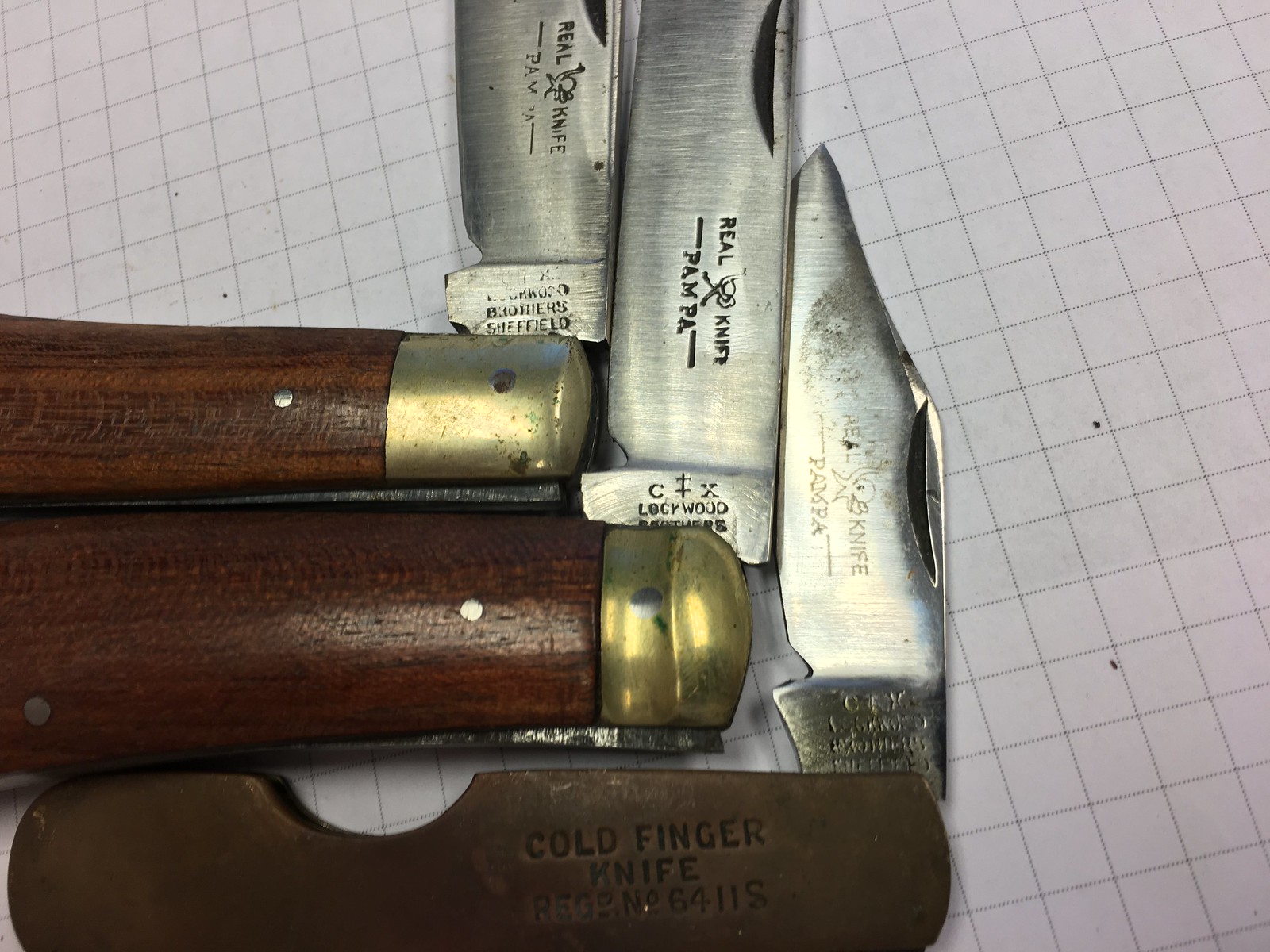A high-quality photograph captures a close-up of three vintage pocket knives, meticulously arranged at a 90-degree angle on a piece of white grid paper. The handles of the top two knives feature dark chocolate wood with brass end caps, while the bottom knife sports a cooler brown metal handle with a distinct divot and a slightly dirty finish. Each blade, aged and varying in size, is engraved with "Real Knife Pampa" and a saber sword design. Notably, the bottom knife also bears the text "Cold Finger Knives." Despite their age, the detailed engravings and the unique characteristics of each knife's handle are clearly visible. The knives, likely between 50 to 100 years old, each tell a story of craftsmanship and history, further identified by additional inscriptions such as "CX Lockwood" and "Sheffield."